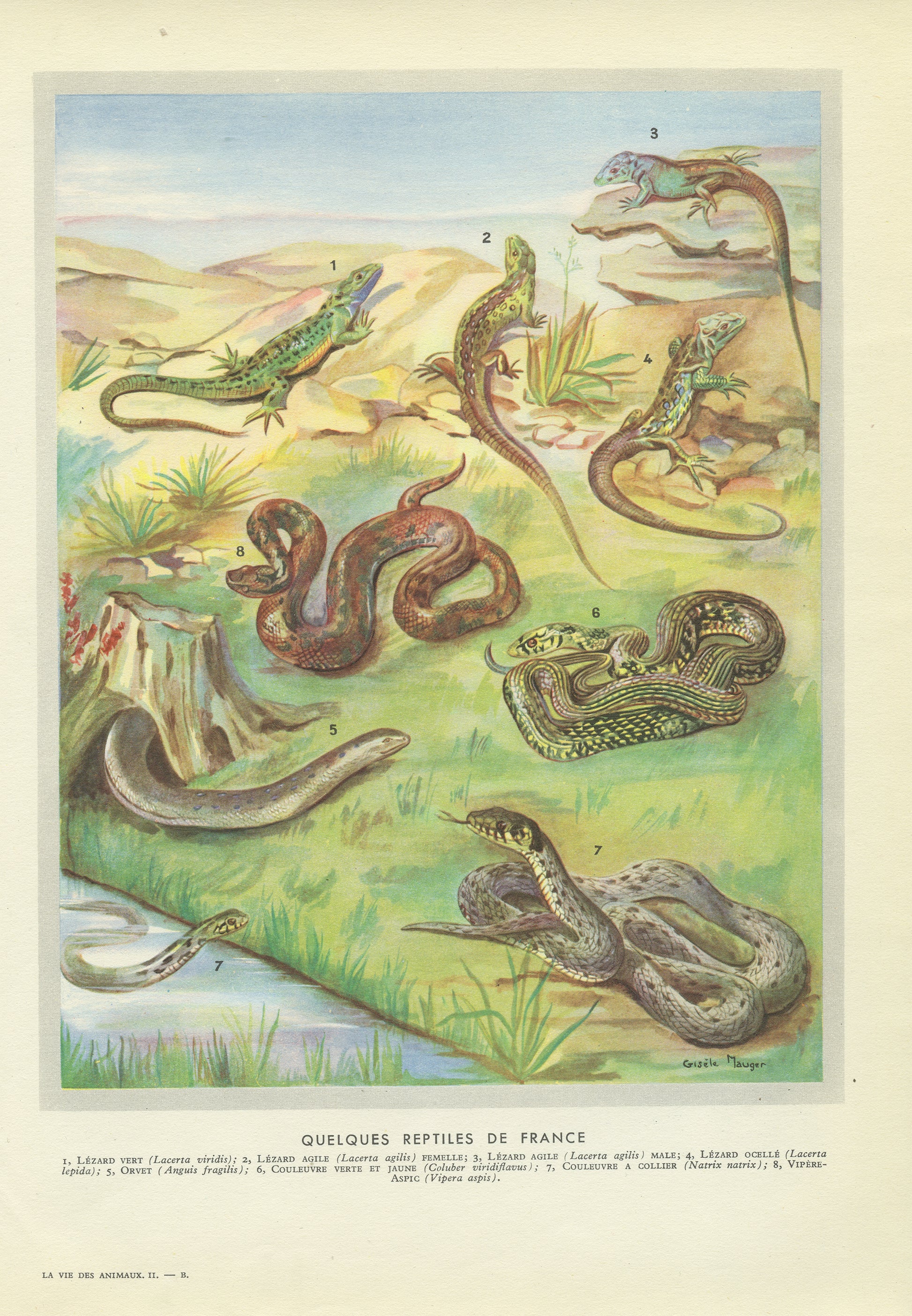This detailed illustration appears to be a colored plate from a textbook, specifically depicting reptiles of France, as indicated by the label "Qualicus, Reptiles of France" at the bottom. It features a variety of lizards and snakes, each numbered and described in a visually compelling manner. The background page is cream-colored, bordered lightly in gray. 

At the top of the image, four lizards are perched on rocks, each numbered 1 through 4. Lizard number 1 is at the highest position, with lizard number 2 next to it, seemingly gazing into the distance. Below them, lizard number 3 sits atop a rock, and lizard number 4 is positioned lower, appearing alert.

In the middle portion, there are four larger snakes, each coiled and distinct in appearance. Snake number 5 is gray, while snake number 6 is spotted green. Snake number 7, also green-spotted, appears to be emerging from a water body, and snake number 8, maroon-red, looks poised to strike.

At the bottom left, a water snake labeled number 7 is visible with its head protruding from the water. Nearby, another snake is seen emerging from the root of a tree.

All these reptiles are thoughtfully arranged to convey the diverse habitats they occupy, with lizards predominantly on rocks and snakes scattered among water, grass, and tree roots. Each reptile's number corresponds to additional descriptive text likely found at the bottom of the page, offering further insights into their identification and characteristics.